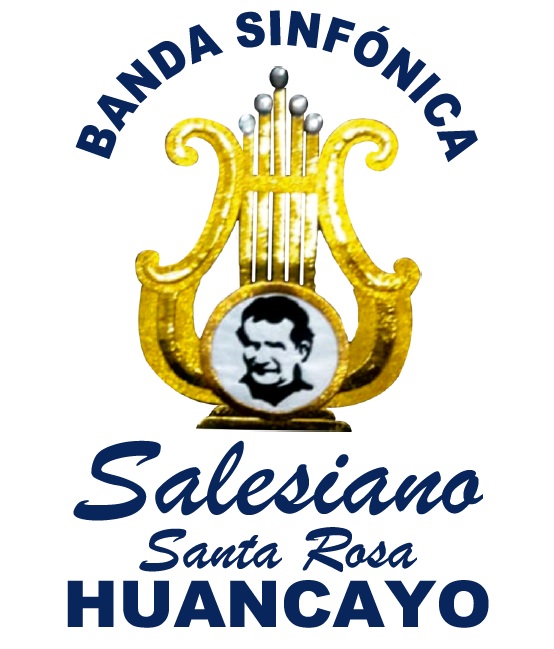In this image, there is a logo centered against a solid white background, resembling a sign or poster associated with a Spanish-speaking area. At the top, blue text in all capital letters curves in a semicircle and reads "BANDA SINFÓNICA." Below this text, a shiny, golden harp-like instrument is prominently displayed. This instrument features scrolls on both sides and silver ball tips, giving it a trophy-like appearance. In the center of this golden trophy is a circular frame enclosing a black and white sketch of a man's face. Beneath the instrument, the text reads "SALESIANO," with additional lines of text below stating "Santa Rosa" and "HUANCAYO" in all capital letters. The overall style has a graphic design quality.